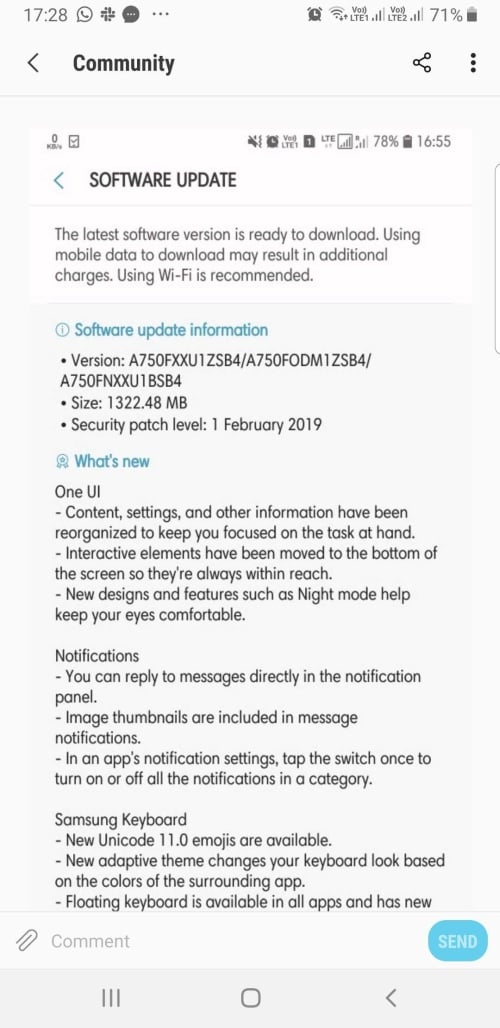This is a detailed screenshot of a smartphone displaying a webpage related to a software update. The timestamp reads 17:28, and the status bar includes a phone icon, an alarm icon, a Wi-Fi icon, and a battery level indicator showing 71% with LTE1 connectivity. Prominently at the top, a left-facing arrow labeled "Community" appears in black text.

Below the "Community" label, there is a section titled "Software update." This section informs the user that the latest software version is ready for download. It advises that using mobile data may result in additional charges and recommends using Wi-Fi.

The software update information is detailed through three bullet points:
1. **Version**
2. **Size**
3. **Security patch level**

Following the bullet points, there is a "What's new" section, detailing updates and improvements which include:
- One UI
- Content settings and other information
- Notifications
- Samsung Keyboard

At the bottom of the screen, there's a text box for entering comments and a send button. The bottom border of the screen features three vertical lines for additional options, a home button, and another left-facing arrow for navigation.